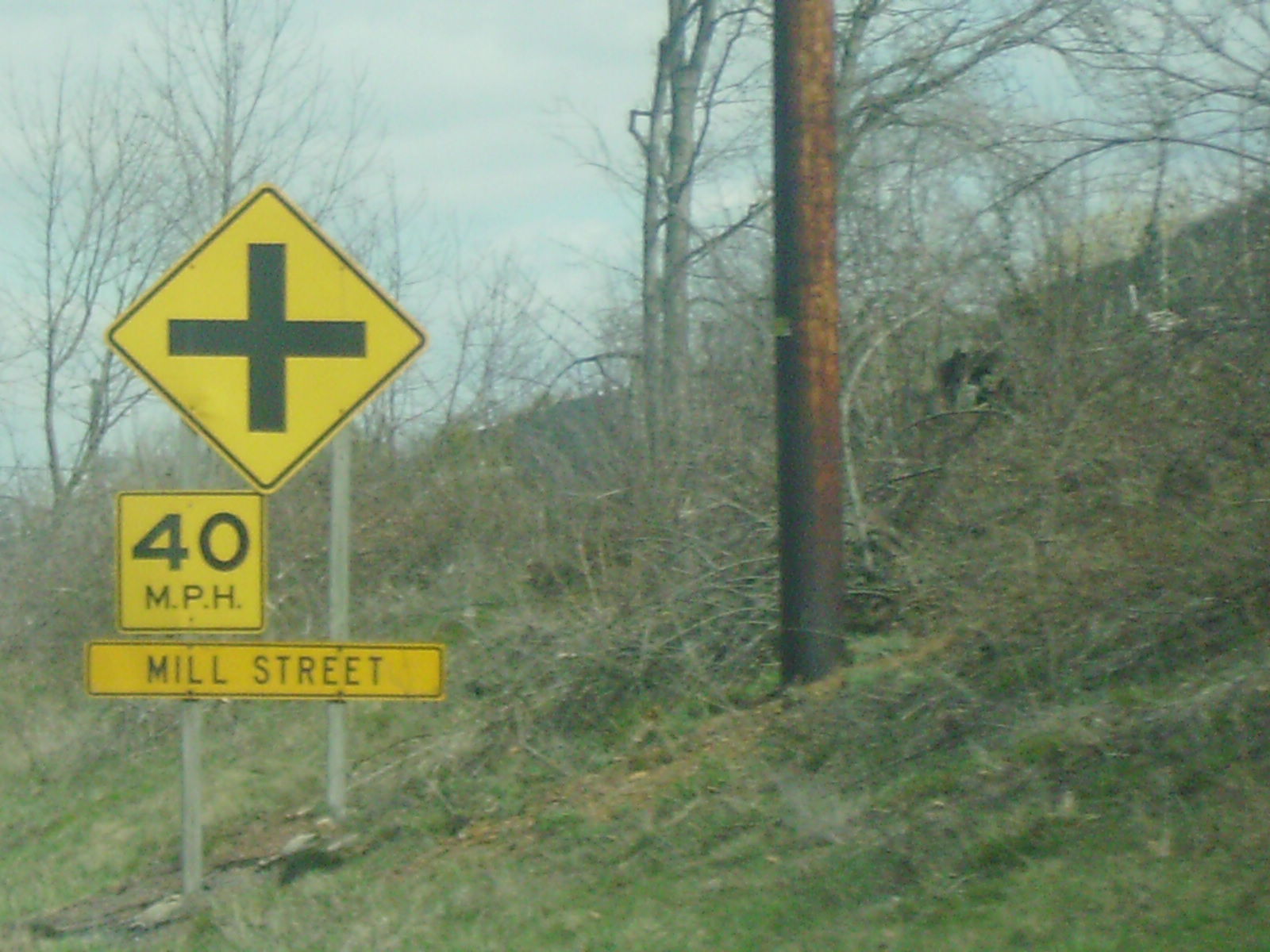This photograph captures a somber winter scene along a roadside that climbs up a steep embankment. The embankment is dotted with barren trees, their branches stripped bare of leaves, signaling the transition from autumn into winter. The landscape is enveloped in a lifeless, gray hue, giving the impression of cold and desolation.

In the center of the image stands a tall structure that draws immediate attention. At first glance, it resembles a large tree trunk, but it could also be a telephone pole. This pole exhibits a dark, rusty brown color, possibly due to weather-induced discoloration, suggesting it might be made of either aged metal or tarred wood.

To the left of this pole, a series of street signs are mounted on metal posts. One sign, with a rectangular shape, discloses the street name as "Mill Street." Another is a square, yellow sign with black lettering, indicating a speed limit of 40 miles per hour. The largest sign is diamond-shaped, featuring a bold, black cross, alerting drivers to an upcoming major intersection or four-way stop.

The sky overhead is a blank, overcast gray, devoid of any sunlight, contributing to the chilly and bleak atmosphere of the scene. The entire composition evokes a sense of quiet and stillness, characteristic of a cold, wintry day.